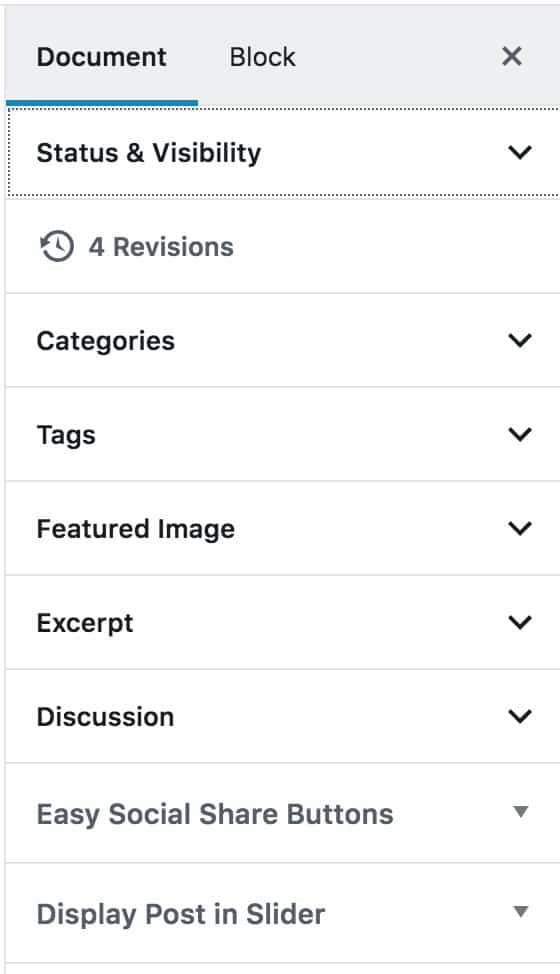A meticulously captured photograph of a cell phone screen displaying a document editing interface. At the top of the screen, within a gray header, there are two tabs labeled "Document" and "Block", underlined by a blue line. Below this header is a section titled "Status and Visibility," accompanied by a downward-facing arrow resembling an upside-down letter "V". Next is the "Revisions" section, indicated by a clock icon with a circular arrow around it, which lists four revisions but lacks a dropdown arrow.

Further down, the interface features several sections: "Categories," "Tags," "Featured Image," "Excerpt," and "Discussion," all marked with similar upside-down "V" arrows. Additional sections, such as "Easy Social Share Buttons," "Display," "Post," and "Slider," are represented with downward-pointing triangle arrows, giving the impression of arrows aimed downward. In the upper right-hand corner of the gray box, there is an 'X' icon, situated next to the "Document" and "Block" tabs, neatly closing the interface view.

This detailed view highlights the comprehensive array of options available for editing and customizing the document's settings, visibility, and content features.